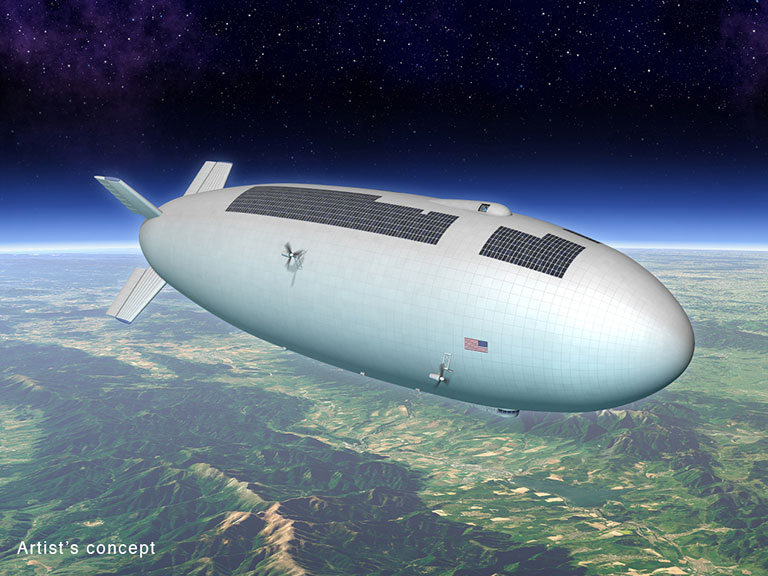This detailed illustration showcases a futuristic blimp or zeppelin prominently centered in the image, denoted as an "artist's concept" in white lettering in the bottom left-hand corner. The blimp, which is predominantly white with segmented paneling, features a small backward American flag on its side along with intricate metal detailing. At the top of the blimp, a series of solar panels are depicted, interrupted by a central gap and a protuberance likely designed for human occupancy. Four propellers are mounted at the rear of the blimp. 

The blimp appears to be traveling at a high altitude, just above or at the edge of Earth's atmosphere, suggested by the transition from the detailed rendering of green and dark green mountains and tanned fields below to a gradient sky that shifts from light blue to medium blue, and ultimately to a black night sky dotted with stars. This positioning creates an effect where the blimp appears to be hovering on the cusp between the troposphere and outer space, emphasizing both its cutting-edge design and functional capabilities. Tail fins can be spotted to the left of the blimp, contributing to its elongated, oval, or bullet-shaped structure.